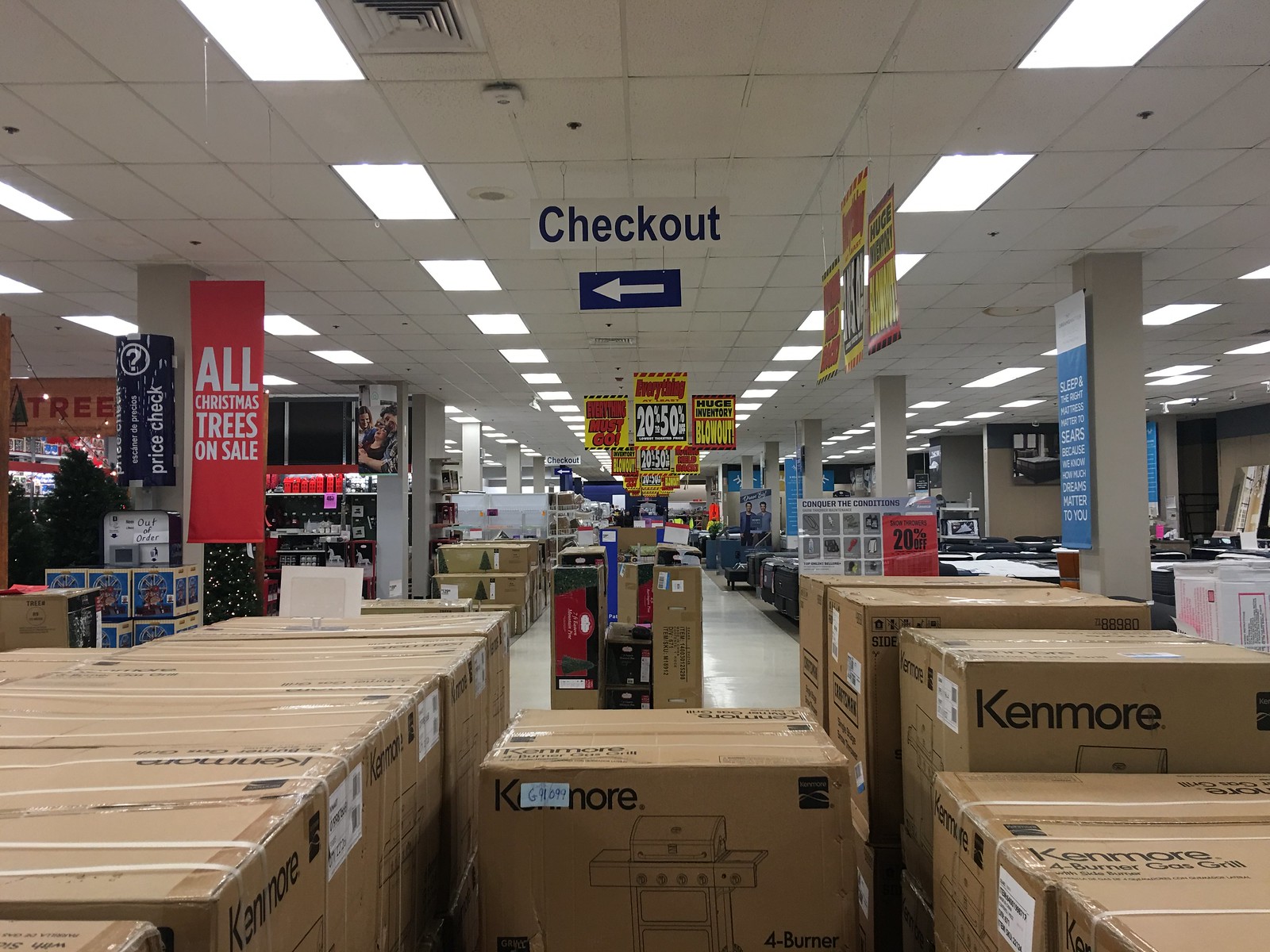The photograph captures the bustling interior of a liquidation store. Central to the image is a prominent sign announcing a store-wide sale, with discounts ranging from 20% to 50%. In the foreground, a collection of Kenmore barbecues is neatly displayed, ready for eager buyers. The upper middle section features a blue sign with a white arrow directing customers to the checkout area, indicated by the word "checkout" in bold letters. On the left-hand side, another sign catches the eye, advertising a sale on all Christmas trees. Below this sign, a price check scanner mounted on a pole stands ready for use. Several Christmas trees are visible, hinting at a festive theme among the store's discounted goods. Overhead, the store's fluorescent lighting illuminates the scene, casting a bright, even glow across the varied merchandise.